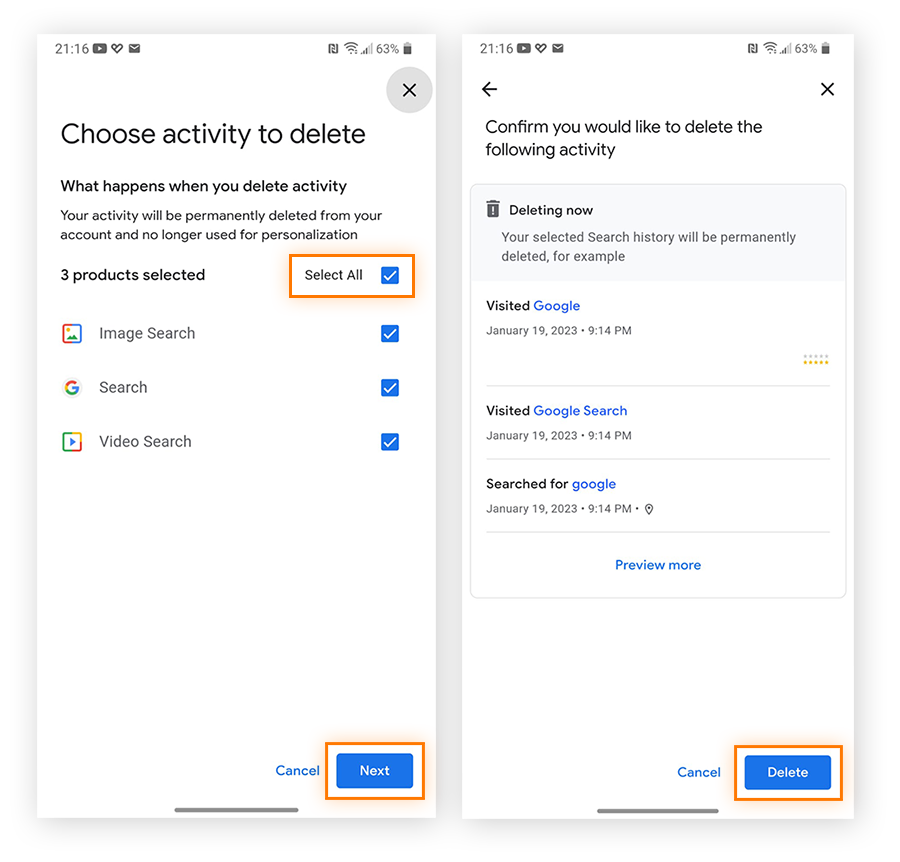The illustration consists of two smartphone screenshots providing step-by-step instructions for deleting activity history. 

**First Screenshot:**
- **Time and Battery:** 21:16, 63% charged.
- **Instructions:** "Choose activity to delete."
- **Warning:** "What happens when you delete activity? Your activity will be permanently deleted from your account and no longer used for personalization."
- **Highlighted Elements:**
  - **"Select All" Box:** Encasing the text indicating three products selected: Image Search, Search, Video Search.
  - **Navigation Options:** "Cancel" or "Next," with the "Next" button highlighted by a green bar.

**Second Screenshot:**
- **Time and Battery:** 21:16, 63% charged.
- **Instructions:** "Confirm you would like to delete the following activity."
- **Action Underway:** "Deleting now, your selected search history will be permanently deleted."
  - **Examples of Deleted Activity:** 
    - Visited Google January 19th, 2023 at 9:14
    - Visited Google
    - Visited Google
    - Search for Google
- **Viewing Option:** "Preview more"
- **Navigation Options:** "Cancel" or "Delete," with the "Delete" button highlighted by a green bar.

This detailed guide clearly illustrates the process and potential consequences of deleting activity history from the account, ensuring users make informed decisions.